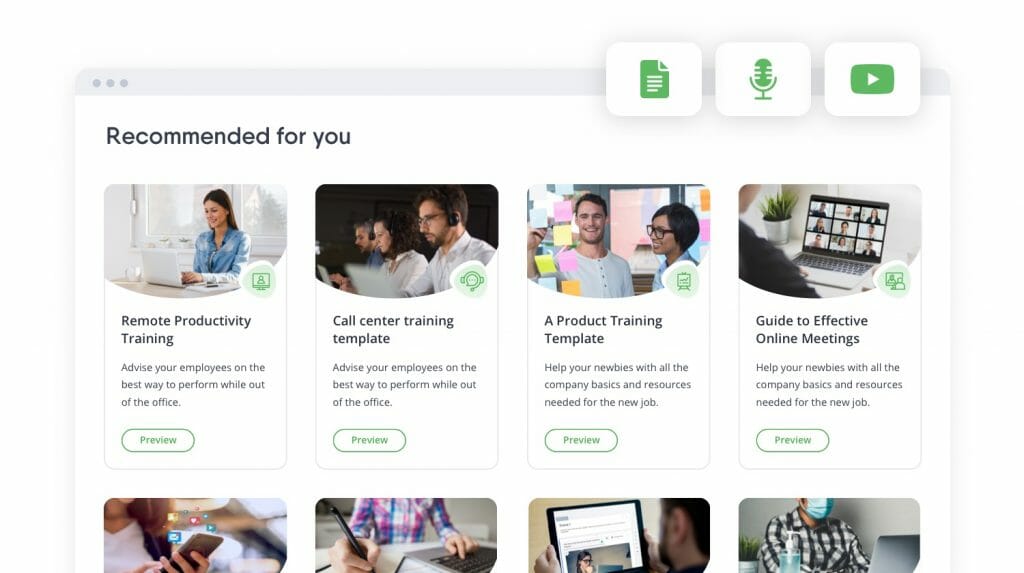This screenshot of a computer screen showcases a user interface with several elements and recommendations. In the upper left corner, a label reads "Recommended for you," while the upper right corner includes three white squares containing icons: one resembling a piece of paper, another depicting a microphone, and the third being a green rectangle with a white triangle pointing to the right, reminiscent of a play button.

Below these icons are four images arranged horizontally. The first image features a woman sitting at a computer with a caption that reads "Promote Productivity Training" or "Remote Productivity Training." The second image shows three individuals at computers in a work setting, captioned "Call Center Training Template."

The third image showcases a man and a black woman looking at sticky notes on a wall, titled "Product Training Template." The fourth and final image depicts someone slightly visible on the left side, facing a computer screen that seems to display a Zoom call; this is captioned "Guide to Effective Online Meetings."

Each of these images has a small green clickable element below it, presumably for accessing further details or content.